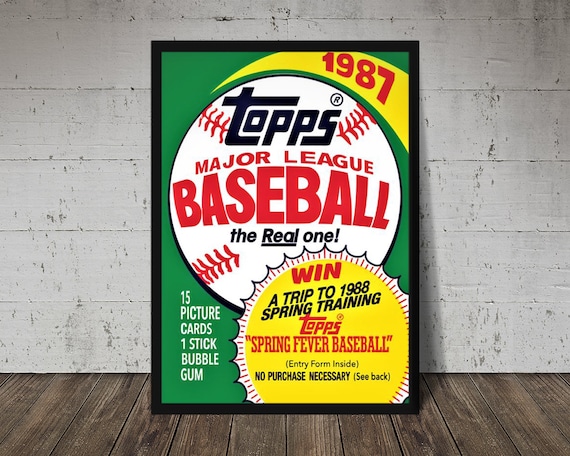The image features a framed poster resembling an enlarged 1987 Topps Major League Baseball card pack. The composition is dominated by vibrant green and yellow hues, with a large baseball centrally placed on the poster. Inside the baseball, in bold red lettering, it reads "Topps Major League Baseball" with "The real one" notably underlined. A yellow stripe above the baseball indicates the year "1987" in red text. Below the baseball, on the left side, white text lists "15 Picture Cards, 1 Stick Bubble Gum." To the right, a stylized yellow sun with red rays and a swooping black outline highlights a prize announcement in red and black fonts: "Win a Trip to 1988 Spring Training." Beneath that, in red, it says "Topps Spring Fever Baseball", followed by the phrases in black text: "Entry Form Inside" and "No Purchase Necessary (see back)." The framed poster is positioned against a worn, off-white wooden wall with gray splotches, resting on a dark wooden floor.